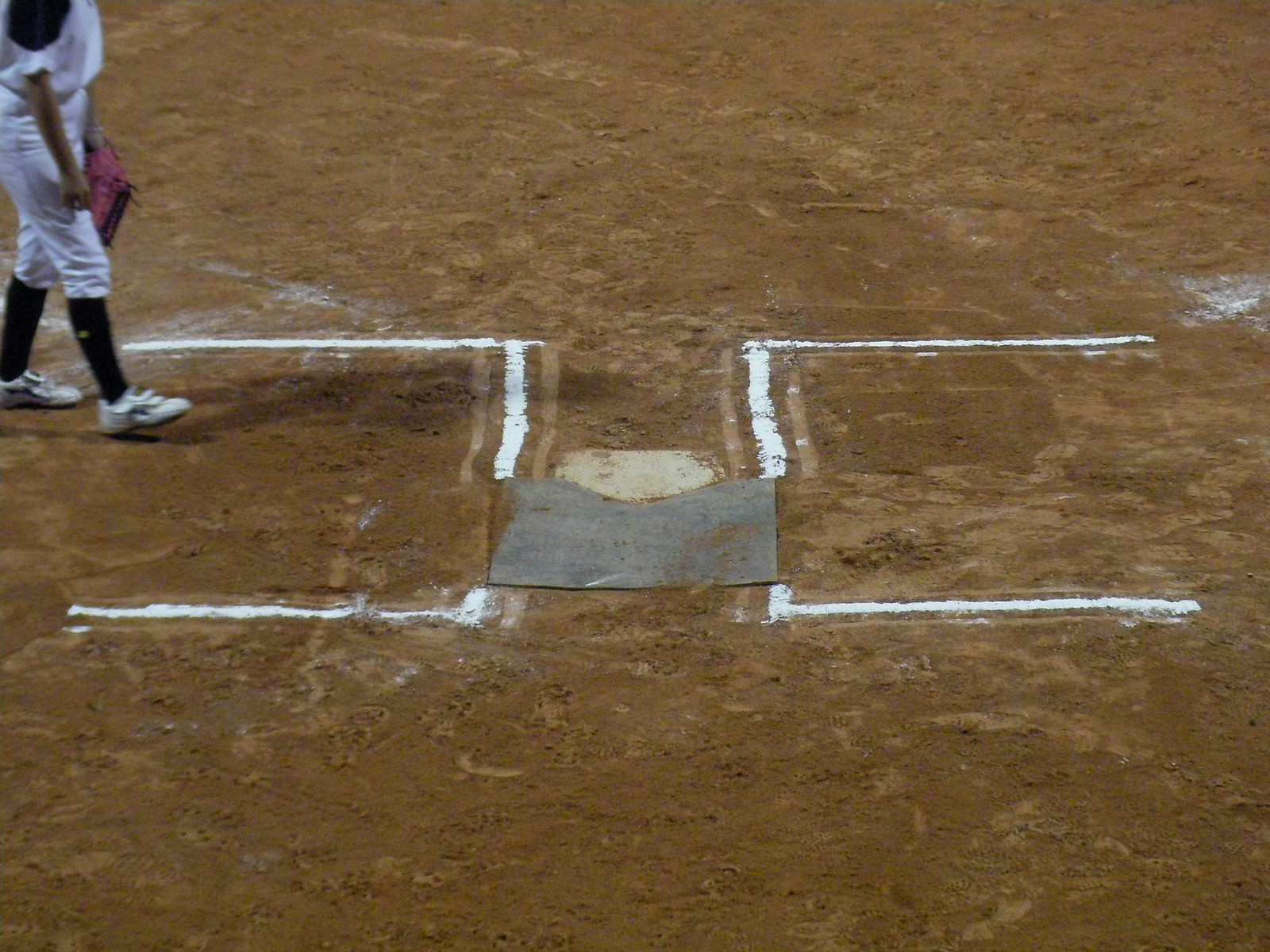The image depicts a small section of a baseball field, primarily focusing on the area around home plate. The ground is made of dark, fine dirt, appearing almost wet due to its dark brown color. In the center, the five-sided home plate is prominently featured, surrounded by additional markings: three-sided chalk lines on either side that form partial squares. A gray, dirty piece lies behind the home plate, adding to the rugged appearance of the area.

In the upper left corner, a baseball player in uniform can be seen. The player wears black high socks, white pants, white cleats, and a white jersey with black shoulders. Holding a reddish-brown baseball mitt, the player's head is cut off by the top edge of the photograph, making only the body visible from the shoulders down. The player appears to be positioned on the third base side, moving towards home plate. The entire scene is slightly blurry and out of focus, hinting at the dynamic motion typical on a baseball field. No other people or objects are visible in the image.